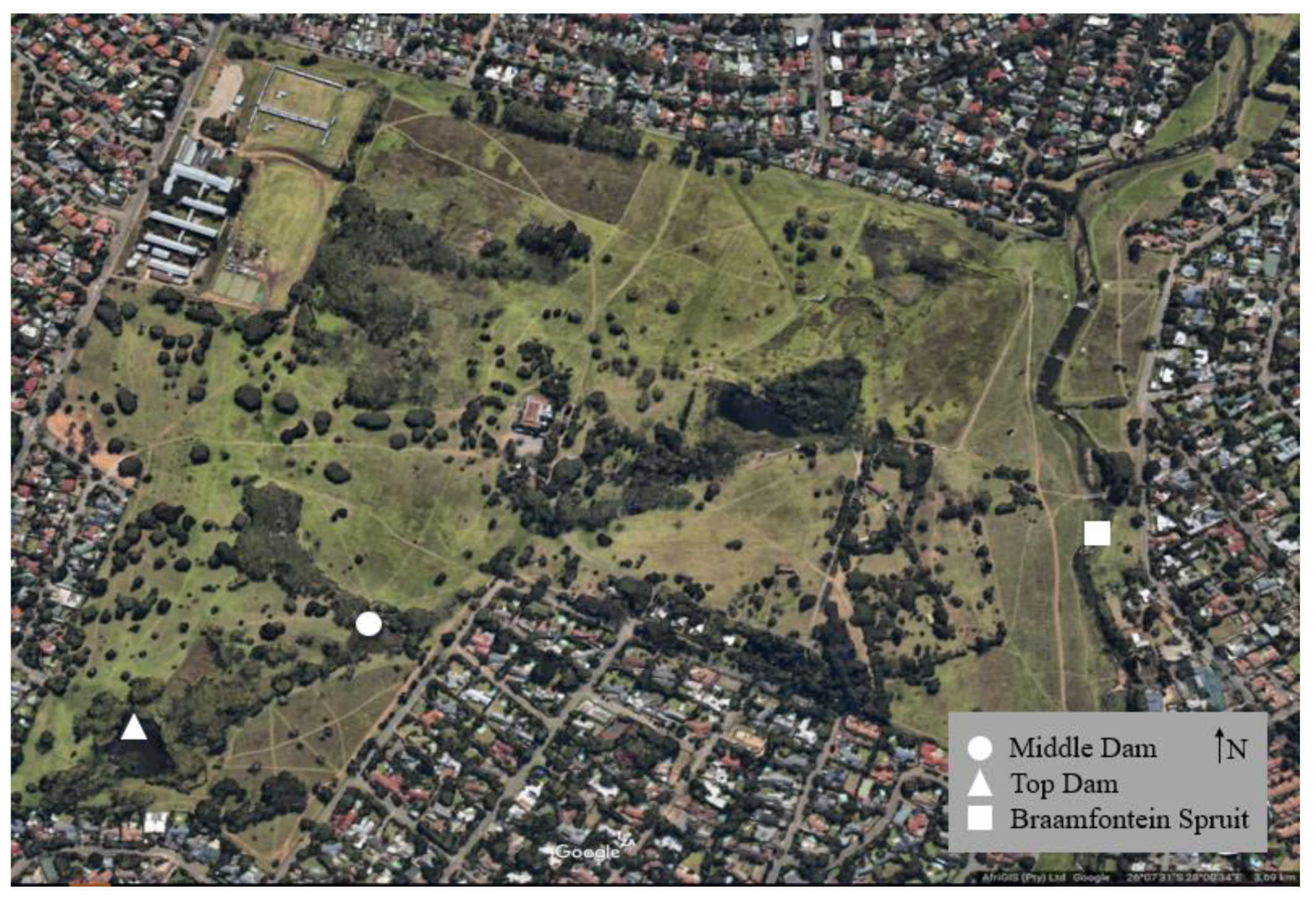This overhead aerial photograph captures a densely populated neighborhood surrounding a central green area, possibly a park or farmland. The green space in the middle is noticeable for its open fields, dotted with trees and intersected by dirt roads or paths. In one corner of this central area, there's a larger rectangular structure, potentially a school or a factory, with an adjacent neatly trimmed field which might be a sports facility.

Encircling the park are grids of compact residential neighborhoods, characterized by varying roof colors—red and gray—and visible driveways with parked cars. The surrounding houses underscore the area's heavy population density, threaded through with numerous roads.

In the bottom right corner of the image, there's a key with symbols labeling significant points: a white circle for the Middle Dam, a white triangle for the Top Dam, and a white square for the Brafontein Spruit. These symbols appear on the map, pinpointing the location of each feature. Also present is a north arrow, giving orientation to the map.